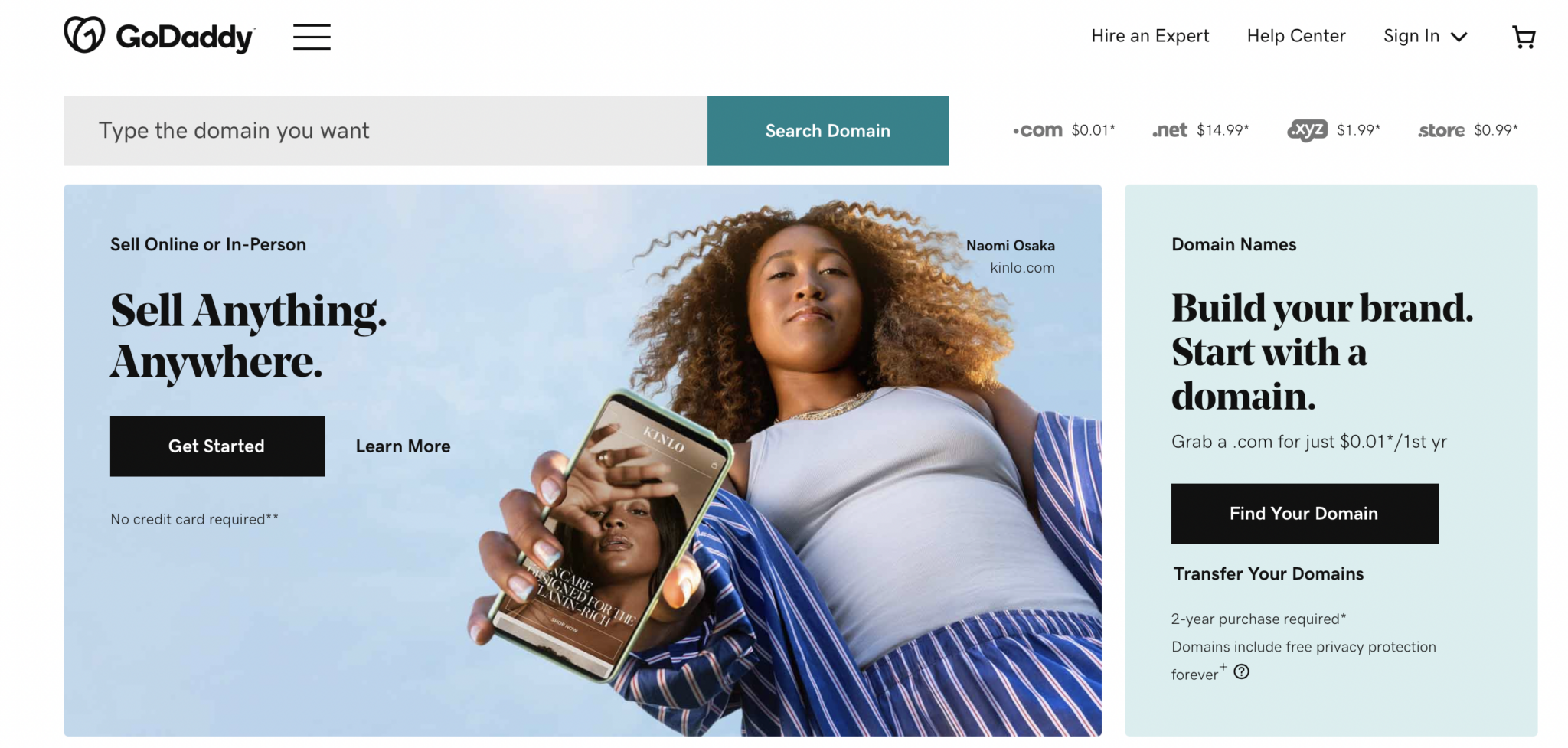The home page of the GoDaddy website is displayed, clearly featuring the recognizable GoDaddy logo in the top-left corner, accompanied by three horizontal bars that indicate a menu. At the very top of the page, there's an intuitive navigation bar that includes options like “Hire an Expert” and “Help Center”, followed by a sign-in button with an accompanying arrow suggesting additional options. 

To the right, an icon of a shopping cart and a search bar prompt users with "Type the domain you want," alongside a prominent "Search Domain" button. Pricing details for various domain extensions are highlighted: .com domains at $0.01, .net at $14.99, .xyz at $1.99, and .store at $0.99.

A prominent banner ad features a young woman holding a phone, promoting the versatility of selling both online and in-person, along with a bold statement: “Sell anything, anywhere.” A striking black "Get Started" button and a "Learn More" hyperlink that emphasizes "No credit card required" are also present. The woman, identified as Naomi Osaka for Kinko.com, is depicted in a white t-shirt layered with a male dress shirt and matching pants. 

Below, another banner urges users to build their brand by starting with a domain name. It promotes grabbing a .com domain for just $0.01 for the first year and includes options for finding or transferring your domain. It also mentions a two-year purchase requirement and highlights that domains include free privacy protection forever. An adjoining question mark offers further details or assistance.